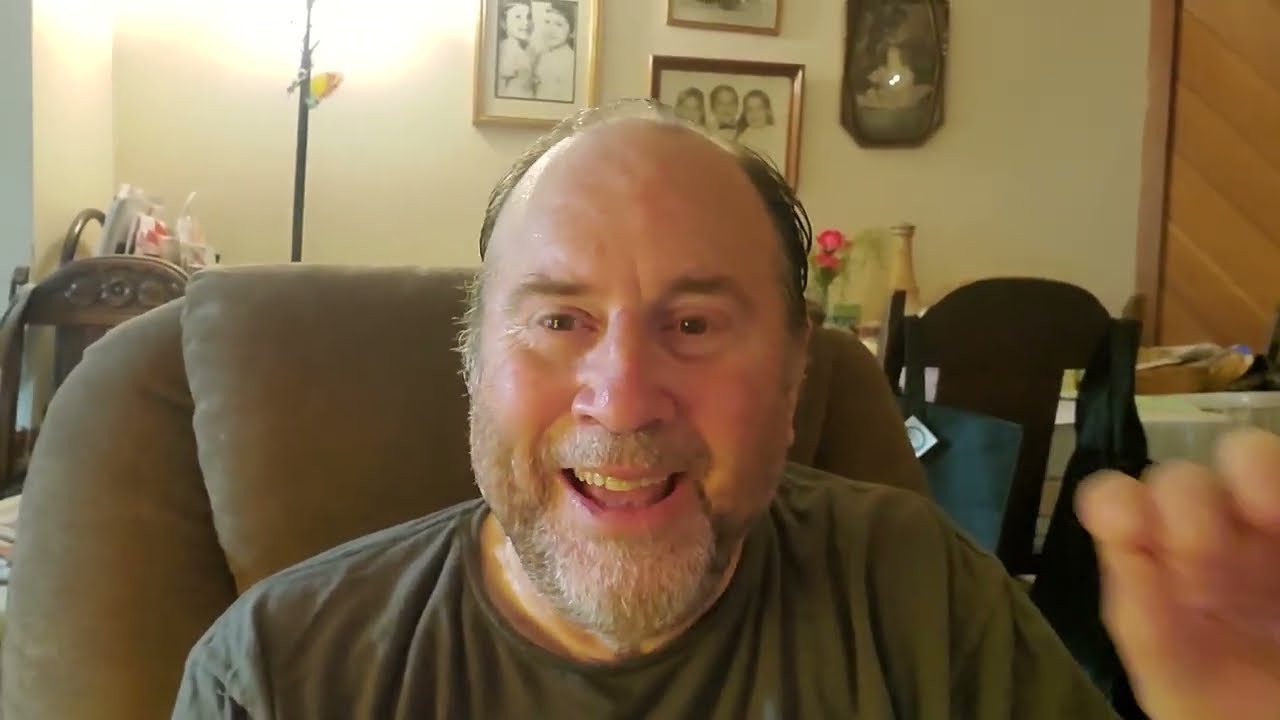The image captures an older white man, likely in his 50s or 60s, taking a casual selfie, possibly from a webcam. Seated directly in a brown suede recliner, the man is centered in the frame and emits a happy demeanor, characterized by his slightly open mouth, revealing his teeth and tongue. He has brown eyes with a joyful glint, a balding head, and neatly cropped gray hair, along with a full beard and mustache that mix gray and a few patches of brown.

He is dressed in a gray shirt, with the image cutting off just above his chest. His left hand is visible in the bottom right corner, poised as if about to wave. The background appears to be his dining room, featuring a dining table with chairs, a floor lamp whose light obscures its shade, and a wall adorned with family photos. Notable objects include pictures of children and an individual by a birthday cake, giving a warm, familial vibe. Additional details in the background include a treadmill on the left, cluttered with trinkets, and a wooden panel wall on the right, adorned with a bottle of wine or champagne and a couple of pink roses, suggesting a cozy, lived-in space.